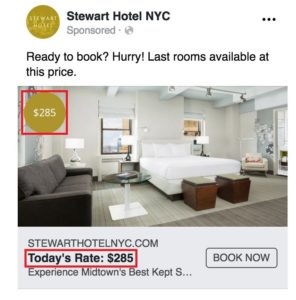A detailed descriptive caption for the image could be:

"This is a screenshot of a mobile advertisement for the Stewart Hotel in New York City, appearing on a platform like Instagram or Meta. The ad features a crisp and inviting image of a well-furnished hotel room. Below the image, the ad prominently highlights the room rate of $285, encased in a bold red box for emphasis. This rate is specifically marked as 'Today's Rate,' which is written in bold text directly underneath the room image and also highlighted with a red box. At the top of the advertisement, a compelling call-to-action reads, 'Ready to book? Hurry! Last rooms available at this price,' urging potential guests to take immediate action. Additionally, a link is provided for users to book a room at the stated rate of $285."